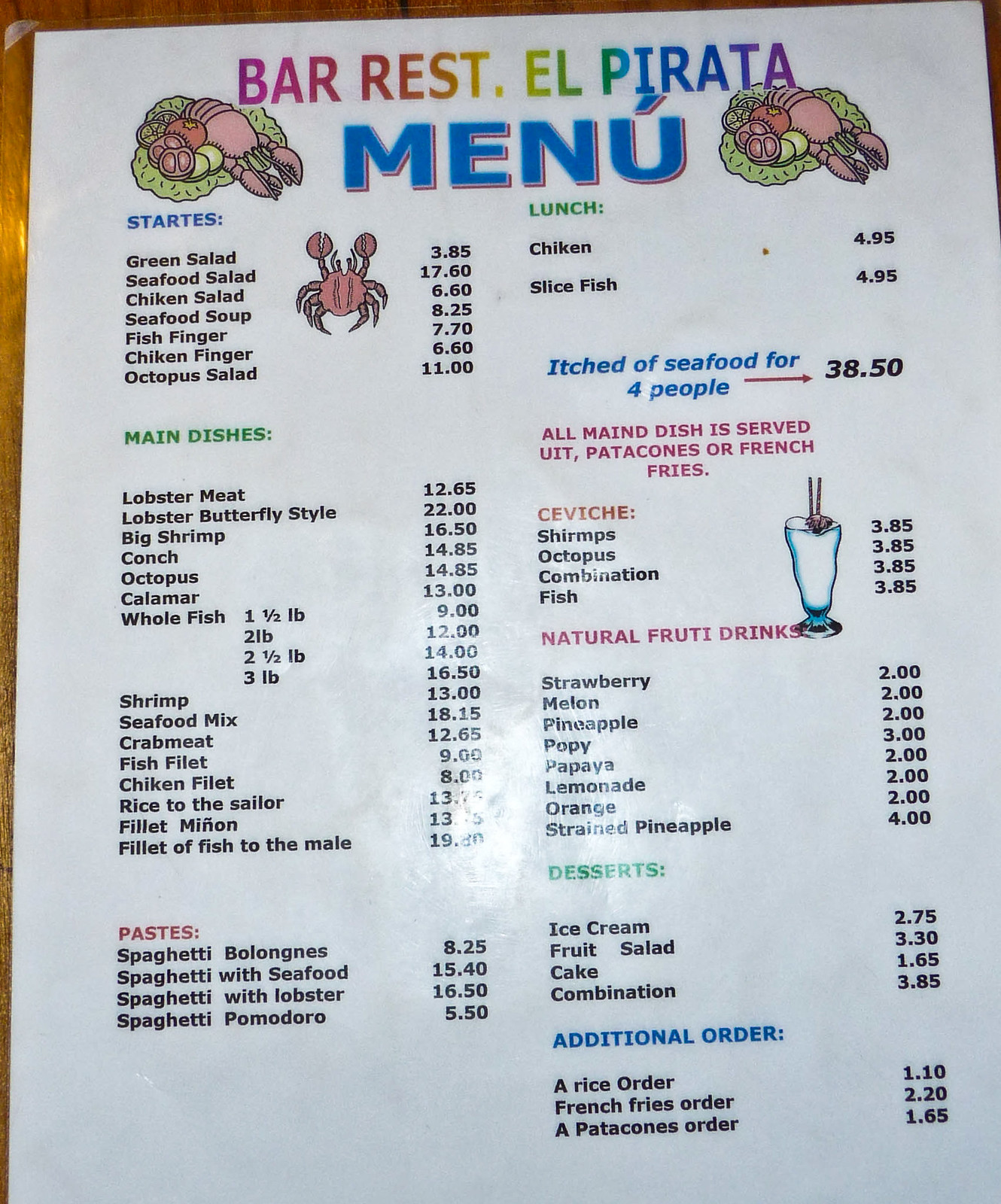This is a detailed photograph of a laminated menu from "Bar Rest El Pirata." The menu is printed on an 8.5 by 11-inch white paper, featuring the restaurant's name "El Pirata" in vibrant rainbow colors at the top. Below the header "Menu," which is in blue, there are illustrated drawings of lobsters on lettuce leaves, garnished with tomatoes and cucumbers, symmetrically placed on either side.

The menu itself is divided into several sections, including starters, main dishes, pastas, and desserts. The starters list items such as seafood soup, chicken fingers, and octopus salad. Main dishes offer a variety of seafood and meat options, including lobster meat, lobster butterfly style, conch, octopus, chicken, and beef.

For beverages, there are natural fruit drinks available in flavors like strawberry, melon, pineapple, and papaya. Dessert options include ice cream, fruit salad, cake, or a combination thereof. Sides available with the meals are rice, french fries, or pasta.

The menu is placed on what appears to be a light-colored wooden table, adding a rustic touch to the overall setting. This detailed depiction gives a comprehensive view of the offerings at Bar Rest El Pirata, suggesting a diverse menu with an emphasis on seafood.